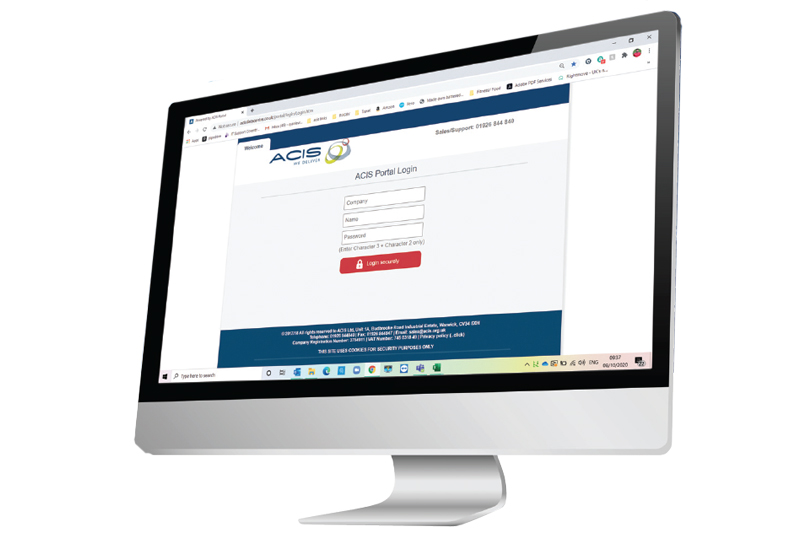A computer monitor displays a web page titled "ACIS Portal Login" prominently at the center. The interface asks for a company name and password, specifying the password requirements as "intercharacters, 3 plus character 2 only." The login prompt also emphasizes the need for secure login practices. The backdrop of the page is stark white, providing a clean and professional look, while thin blue borders mark the top and bottom of the screen, lending a subtle yet distinct frame to the web page.